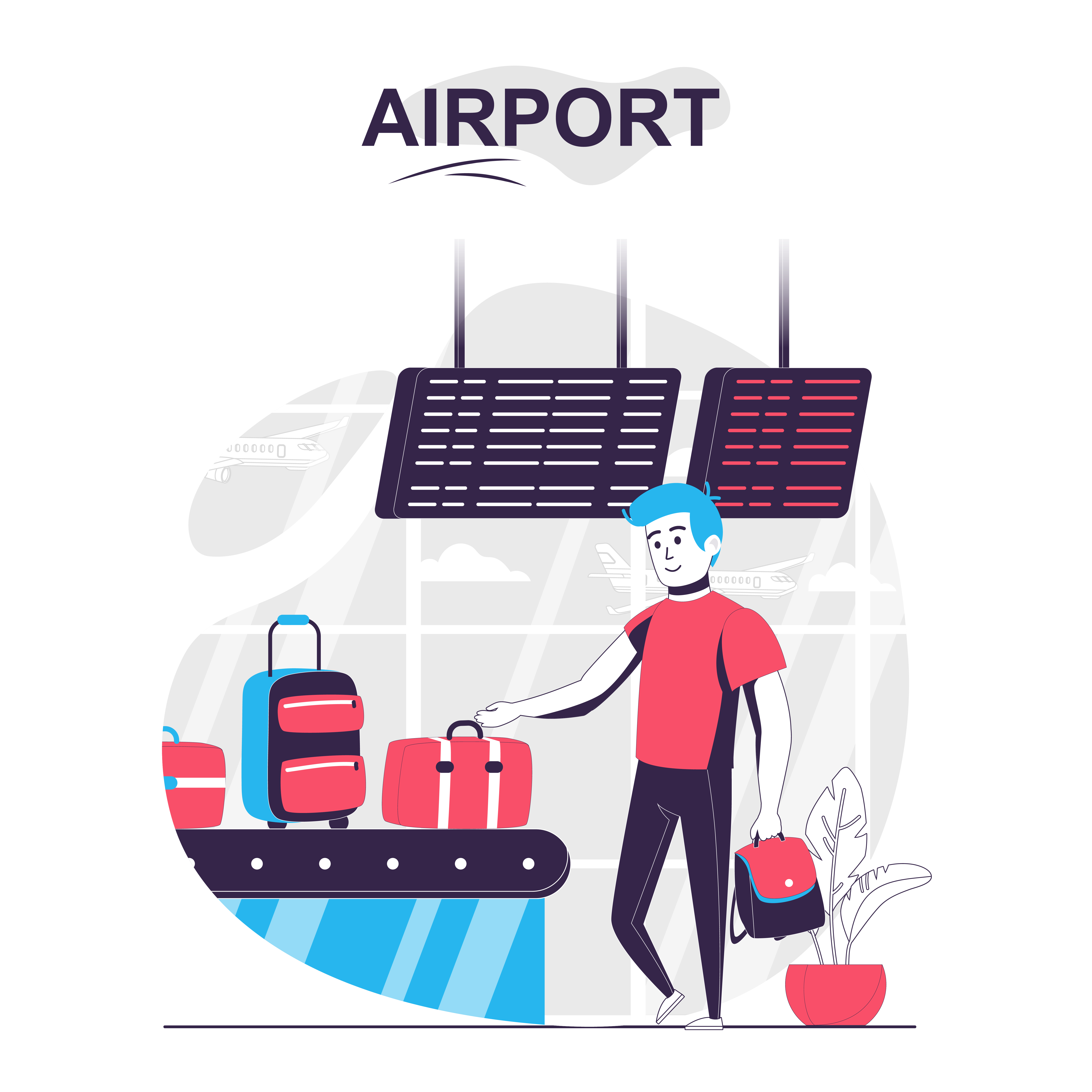In this digital cartoon image set in an airport, a simplistic, stylized man with blue hair is depicted picking up his luggage. The image features a muted color palette of whites, blacks, reds, blues, and grays. At the uppermost part of the image, the word "AIRPORT" is prominently displayed in black text. Below this, there is a bubble-like frame where the action unfolds against a completely white background.

The man, wearing a red shirt and black pants, is positioned to the right-hand side. He is holding a black and red backpack in one hand and is about to grab a red suitcase with white stripes from a blue conveyor belt, which has a black moving surface. Additional luggage in various shades of red and blue can also be seen on the conveyor belt.

Notable details include a monitor above the man displaying flight information, with the left screen being white and the right screen red. Behind him, a faint outline of a gray, rounded window shows planes flying by. To the right of the man, there is a white potted plant in a red pot. Two squares resembling heaters or vents are situated above his head, one with white lines and the other with red lines. This detailed, minimalist depiction captures the busy, transitional nature of airport travel.